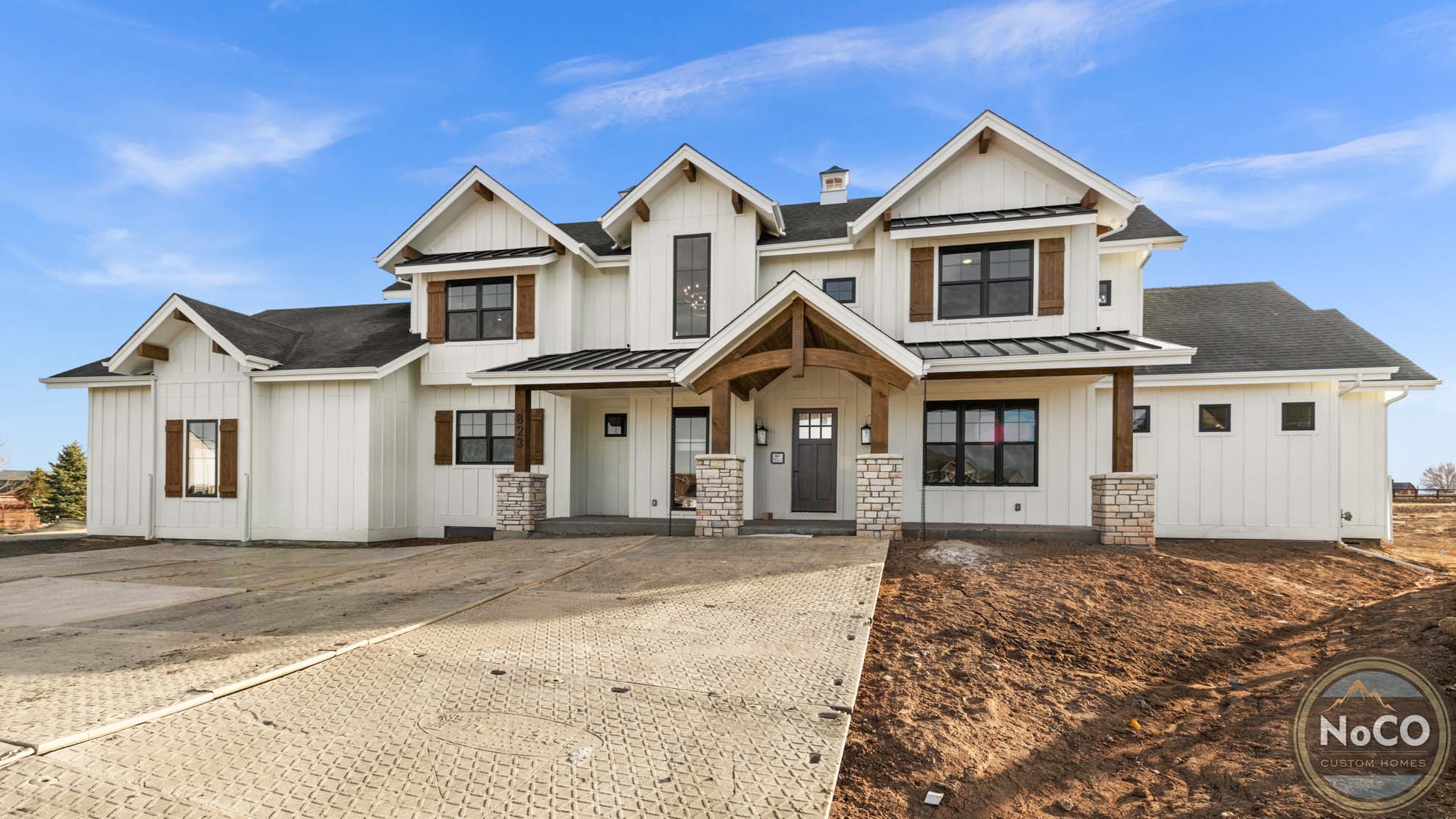This is a horizontal, rectangular color photograph of a large, custom-built house that is currently under construction. The two-story home boasts an expansive and well-structured design, featuring a notable dark-colored front door situated under a gable roof with a small wooden awning and shutters on the windows above. The house is primarily a mix of white and brown tones with wooden elements throughout, adding to its bespoke charm.

The front facade reveals three two-story gables, with an additional single-story section on the side that might serve as a casita or guesthouse. The central portion features a covered porch supported by two white stone columns and matching wood-tone posts, leading to an arched entrance. Above the porch, there's a central roof ornament resembling a small tower with a slanted roof topped in dark gray tin.

A very wide paver driveway extends from the bottom left of the image towards the house, although it transitions into bare dirt directly in front of the garage, indicating that it is still under construction. The right side of the driveway is bordered by reddish-brown dirt, awaiting the installation of a finished lawn.

In the bottom right corner of the image, there's a circular logo displaying "No Co HOMES" with a sketch of a mountain peak, branding the photograph with the custom home builder's mark. This detailed depiction captures a sense of realism, emphasizing the home's sizable and carefully crafted design.